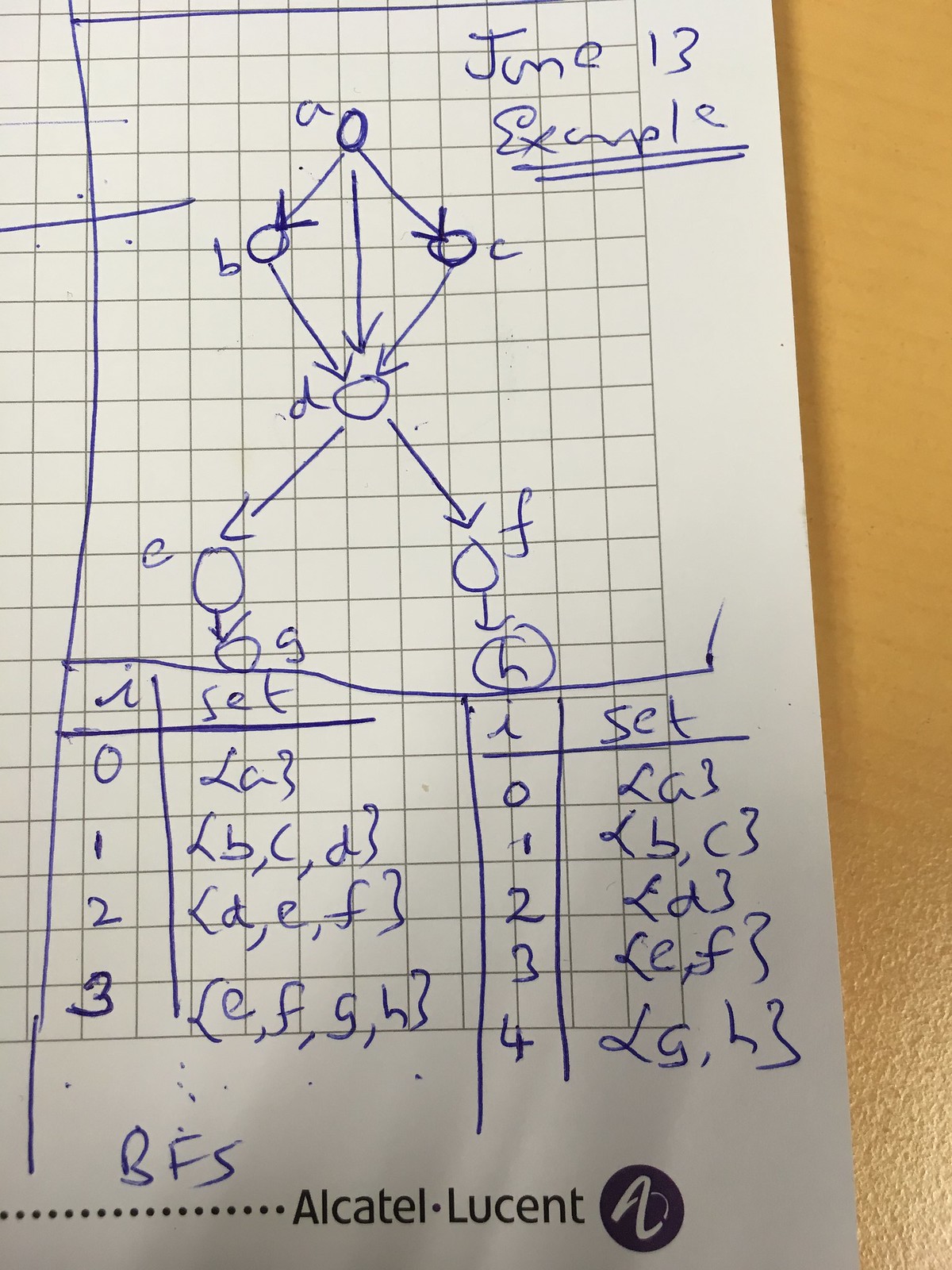The image depicts a detailed hand-drawn diagram on a piece of white graph paper with gray or black gridlines. The graph paper is set against a gold background. The centerpiece of the drawing is a schematic representation of molecular structures, illustrated by circles interconnected with arrows. The circles are labeled sequentially from A to H. 

Beneath the molecular diagram, there are two sections, each labeled with an italic 'I' and the word 'set.' 
- The first section lists:
    - "0" followed by "A"
    - "1" followed by "B, C, D"
    - "2" followed by "D, E, F"
    - "3" followed by "E, F, G, H"
- The second section extends to "4":
    - "0" followed by "A"
    - "1" followed by "B, C"
    - "2" followed by "D"
    - "3" followed by "E, F"
    - "4" followed by "G, H"
    
An annotation at the bottom of the paper reads "June 13th example." Additionally, the bottom of the entire image is labeled "Alcatel-Lucent."